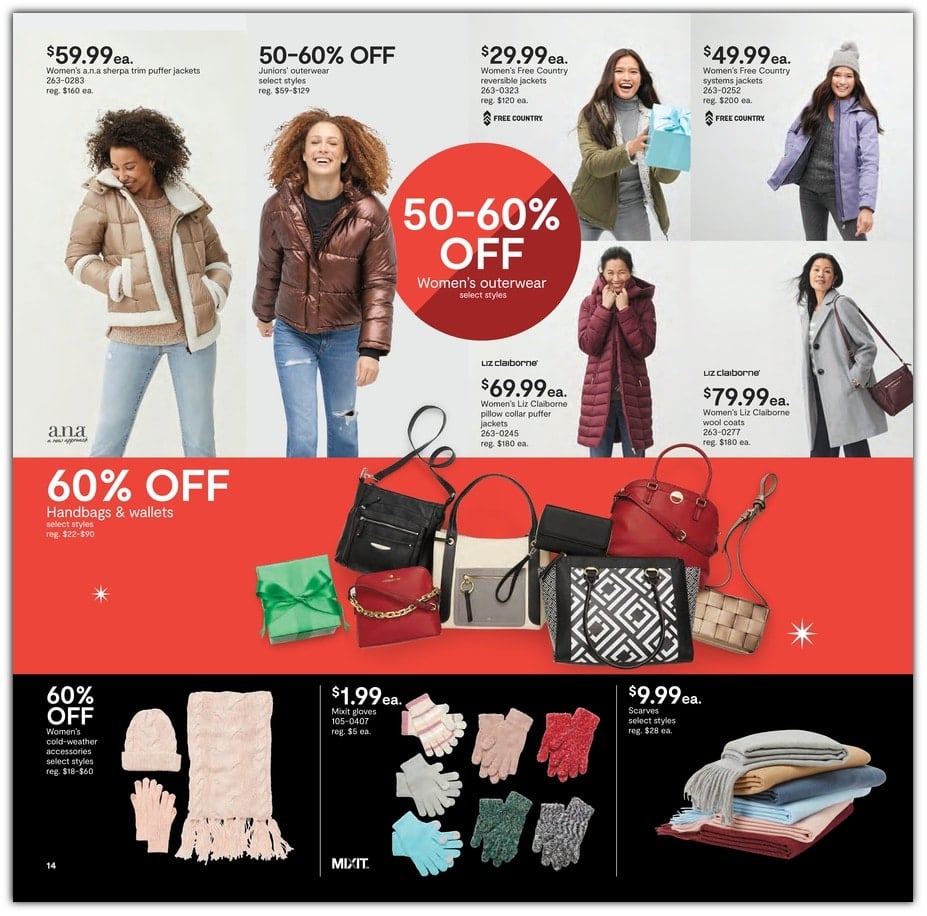This image is a vibrant and detailed clothing catalogue showcasing a variety of stylish female winter apparel and accessories. The catalogue features multiple items with a clear emphasis on outerwear. 

- At the forefront is a cream-colored jacket priced at $59.99, offering a chic and cozy option for the season.
- Next to it is an eye-catching bronze jacket, which is currently on sale with a substantial discount of 50-60% off. The exact styles and final price are selectable and likely vary within this range.
- Also highlighted is a rich green jacket, available for $29.99, presenting an economical yet fashionable choice.
- A striking purple jacket follows, marked at $49.99.
- For those seeking a premium option, a sleek grey jacket is available at $79.99.
- There's also a deep maroon jacket priced at $69.99, adding a touch of warmth and elegance to any winter wardrobe.

Aside from the jackets, the catalogue prominently features accessories:
- Handbags and wallets are showcased with a notable discount of up to 65%, offering a variety of styles and colors.
- Furthermore, gloves and scarves are advertised with a 60% discount, available in an assortment of different hues to complement any outfit.

This appealing spread captures a comprehensive range of winter essentials, ensuring something for everyone looking to enhance their seasonal wardrobe with both style and savings.